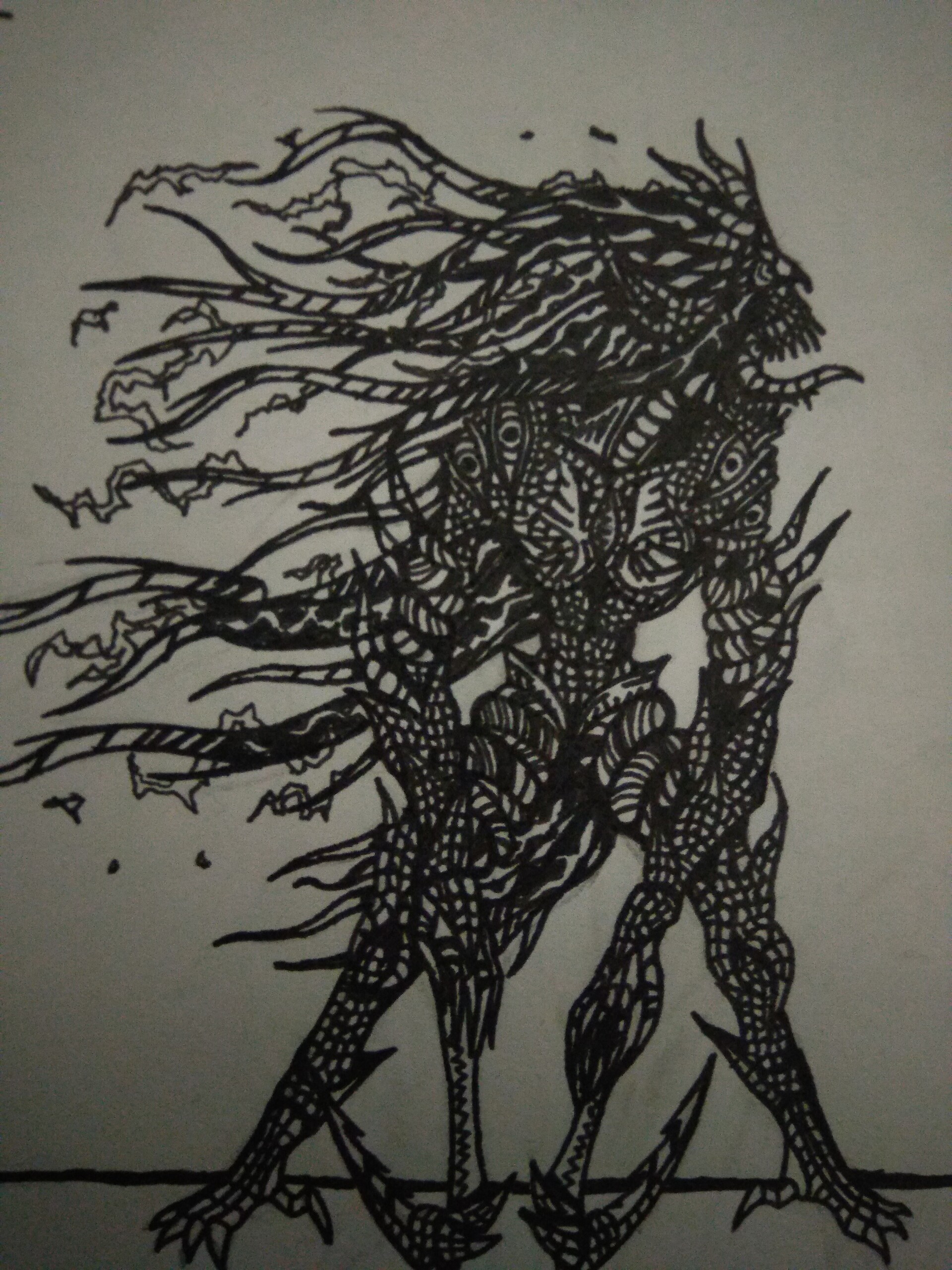The image depicts a detailed black ink drawing of a monstrous creature on a white background. The creature's lower extremities resemble those of a crocodile, with sharp, clawed feet. Its body, appearing to be covered in a mosaic of scales formed by an arrangement of squares and rectangles, suggests a texture similar to that of reptilian skin. Moving upwards, the creature's head features an imposing set of elongated teeth, possibly arranged in dual rows on the upper jaw, unlike the single row seen in humans. Extending from its body are multiple appendages that resemble swinging tails, adding to its menacing and otherworldly appearance.